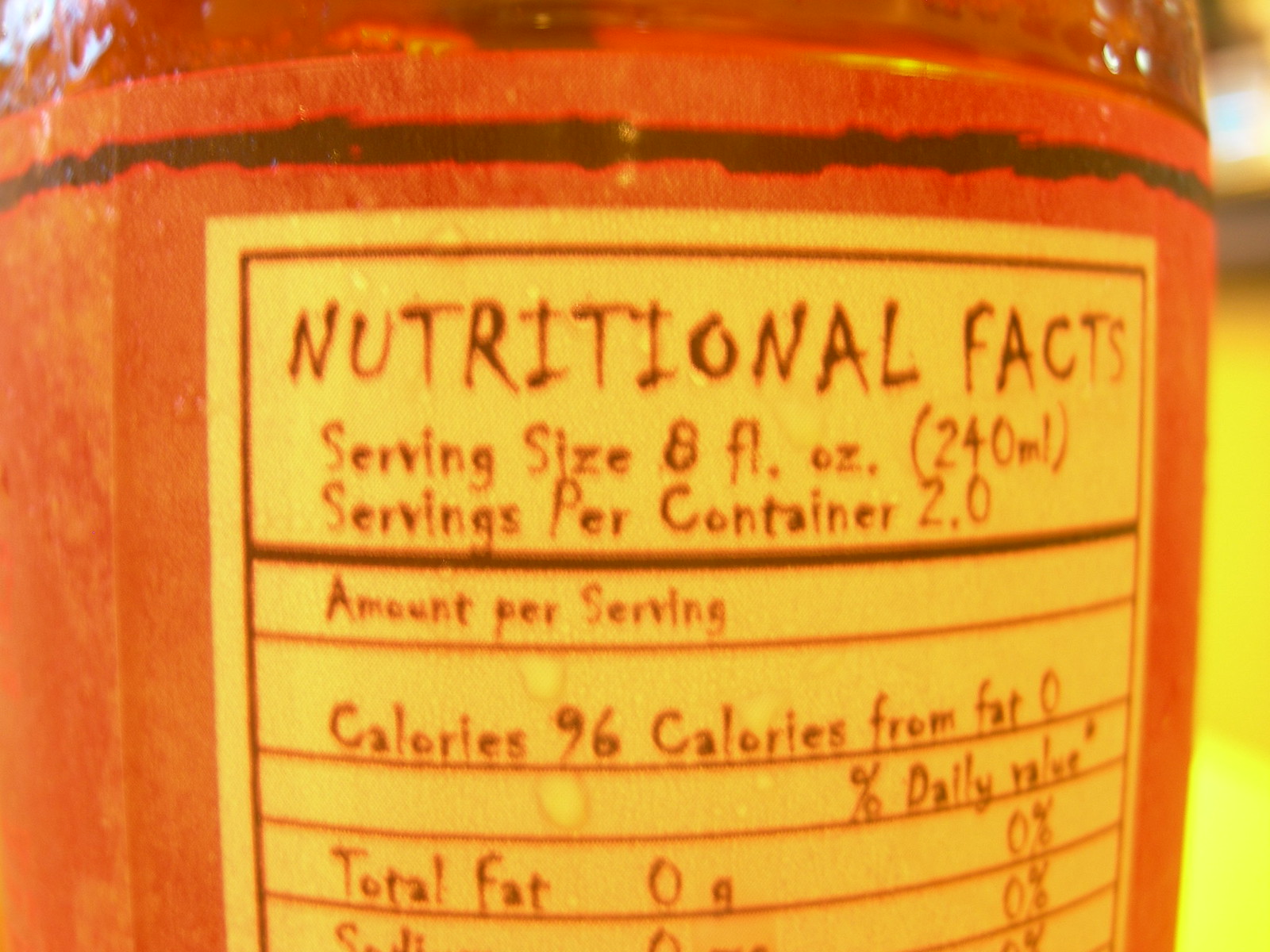The image showcases a close-up of a jar, which appears to be filled with something homemade, accentuated by its rustic, handwritten-like nutritional facts label. The jar features a label with a red background and a black stripe along the top. The nutritional facts label is a light yellowish-gold color, adding to the artisanal feel.

Prominently displayed in capital letters and a blackish-brown hue are the words "NUTRITIONAL FACTS." Beneath this heading, the label details "Serving Size: 8 fluid ounces (240 ML)" and "Servings Per Container: 2.0," followed by a bold black horizontal line. Below the line, the label indicates "Amount Per Serving" and specifies "Calories: 96" with "Calories from Fat: 0." The visible portion of the label also includes "Percent Daily Value" and the beginning of more nutritional information, indicating "Total Fat: 0 grams" and mentioning "Sodium," but the rest of the details are cut off and not fully captured in the photo. This incomplete view adds an intriguing, mysterious quality to the homemade allure of the jar.